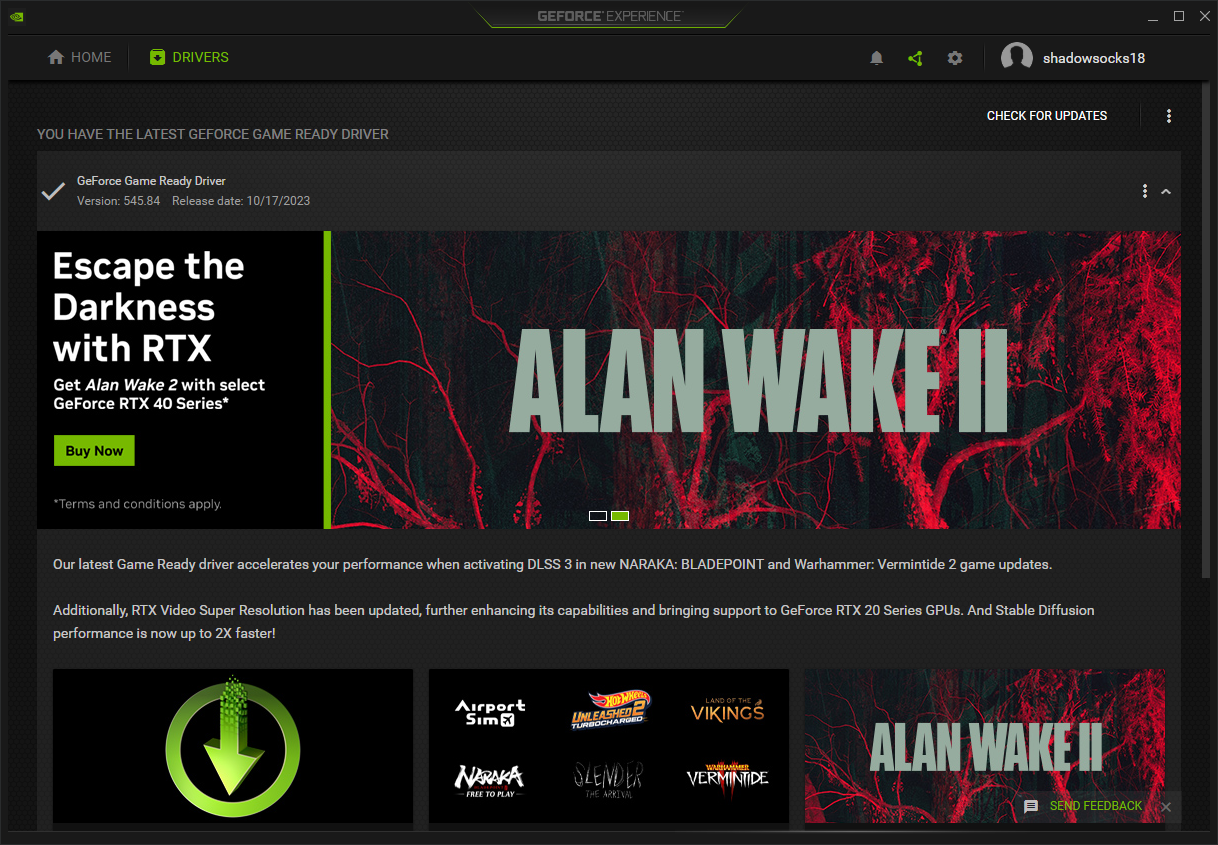Screenshot of the GeForce Experience application showcasing the latest GeForce Game Ready Driver update. The interface features:

- **Top Left Menu:** Tabs labeled "Home" and "Drivers," with "Drivers" highlighted in green indicating the current selection.
- **Driver Information:** Notification stating, "You have the latest GeForce Game Ready Driver," accompanied by a checkmark. The details include the driver version 545.84, released on October 17, 2023.
- **Promotional Banner:** A call-to-action at the center reading, "Escape the darkness with RTX" and mentioning a special offer for obtaining "Alan Wake 2" with the purchase of select GeForce RTX 40 series GPUs. A green "Buy Now" button follows, with an asterisk denoting that terms and conditions apply.
- **Feature Highlights:** Additional information at the bottom highlighting that the latest Game Ready Driver enhances performance for "Naraka Bladepoint" and "Warframe: Heart of Deimos" updates when using DLSS. The update also improves RTX Video Super Resolution for the GeForce RTX 20 series and doubles the performance speed for stable diffusion.

This detailed overview emphasizes the various elements and updates provided to users through the GeForce Experience application.